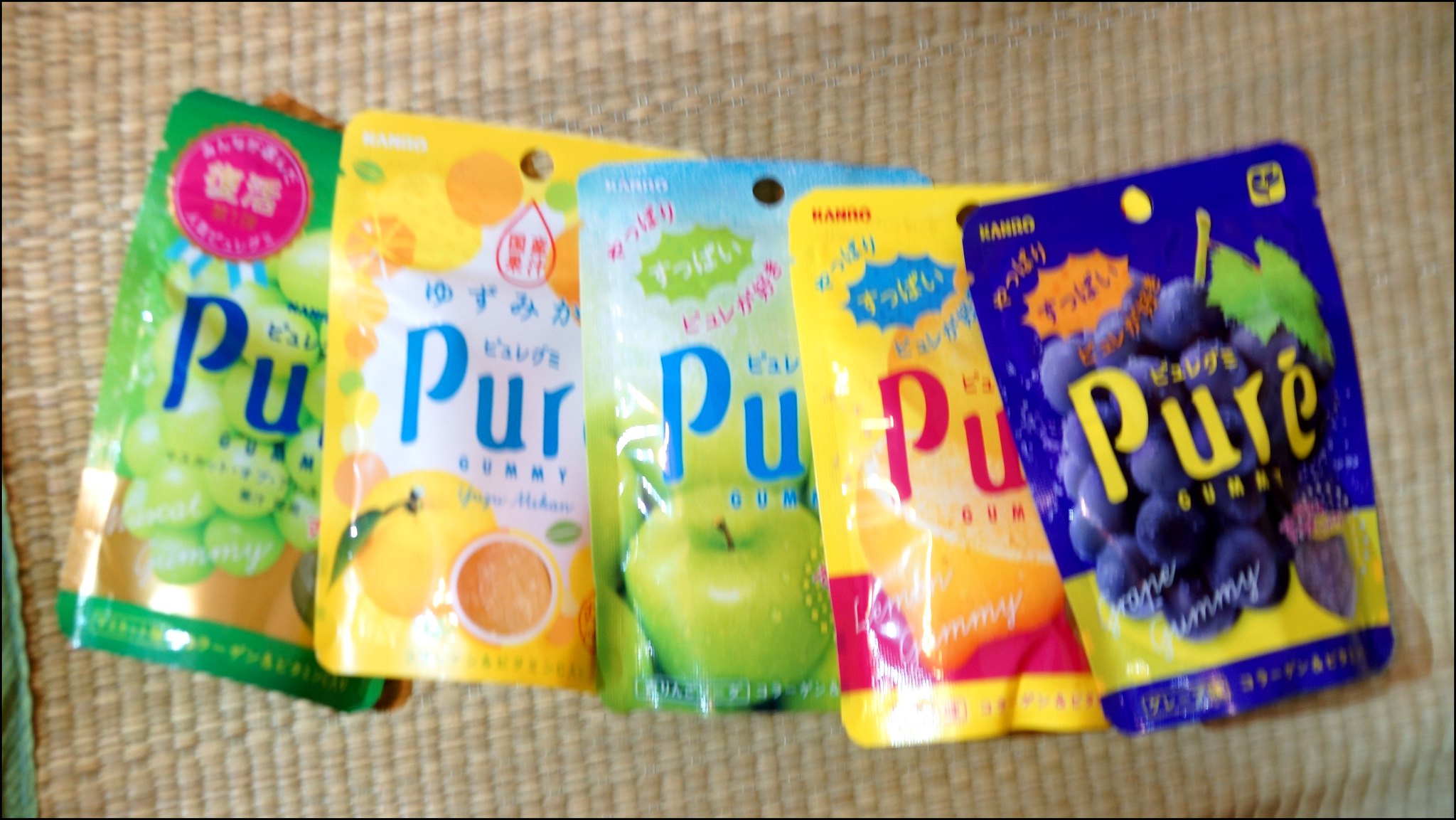In this image, five colorful packets of fruit-flavored items are arranged on top of a light brown, golden tan fabric that resembles a bamboo placemat. There are Japanese characters on the packaging, and each packet prominently features the word "pure" or "puree." 

Starting from the left:
1. The first packet is green, adorned with images of green grapes, and has the word "pure" written in blue.
2. The second packet is yellow, depicting lemons, with "pure" in blue.
3. The third packet has a green and blue background with illustrations of apples, and the word "pure" appears in blue.
4. The fourth packet is a yellowish orange color, featuring an orange, and displays "pure" in red.
5. The fifth packet, on the right, is purple, showcasing purple grapes with a yellow stripe at the bottom and "pure" in yellow letters.

The collection of these vividly colored packets set against the textured fabric background creates a visually appealing arrangement.